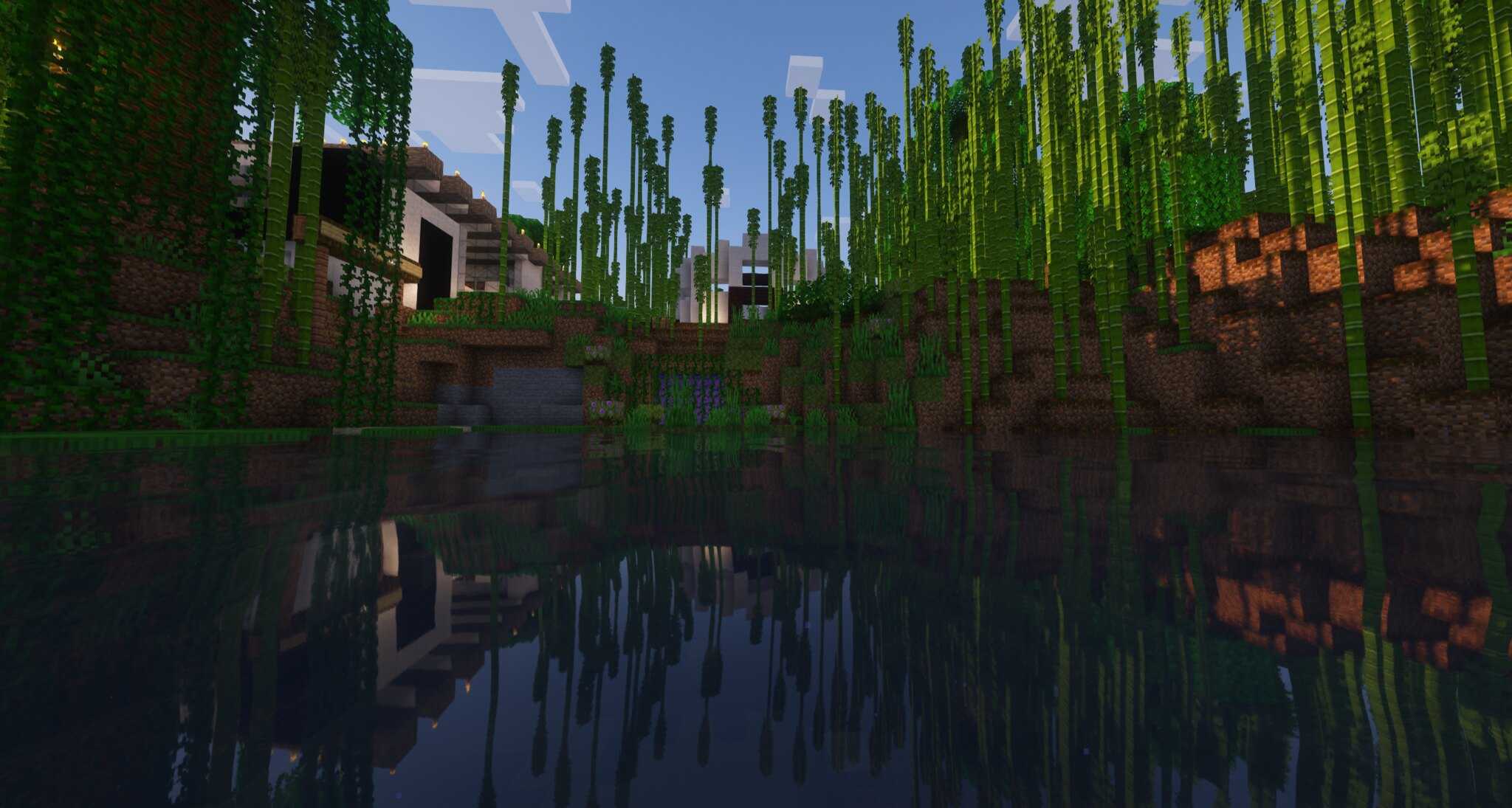This is a screenshot from the video game Minecraft, depicting a serene scene with intricate detail. At the bottom of the image lies a reflective pool of water mirroring the structures above it. The shoreline is elevated and defined by dark brown, block-shaped banks. Sprouting from the shore and cascading downward are green, vine-like structures, devoid of brown trunks, creating a visually striking foliage effect.

On the right, tall, green, tree-like formations rise upwards, adding a sense of natural presence. On the left, steps crafted from brown blocks lead up to a modern-style building. This building is characterized by its white, squared-off architecture, featuring long wooden beams across its flat roof and a dark doorway. 

Further into the distance stands another larger building with a similar angular and contemporary design, maintaining a consistent light gray or bluish-gray color scheme. Above, the sky is a bright blue, dotted with sporadic, squared-off white clouds, adding to the distinctive Minecraft aesthetic. The entire scene is harmoniously reflected in the pristine water below, enhancing the image's tranquil ambiance.